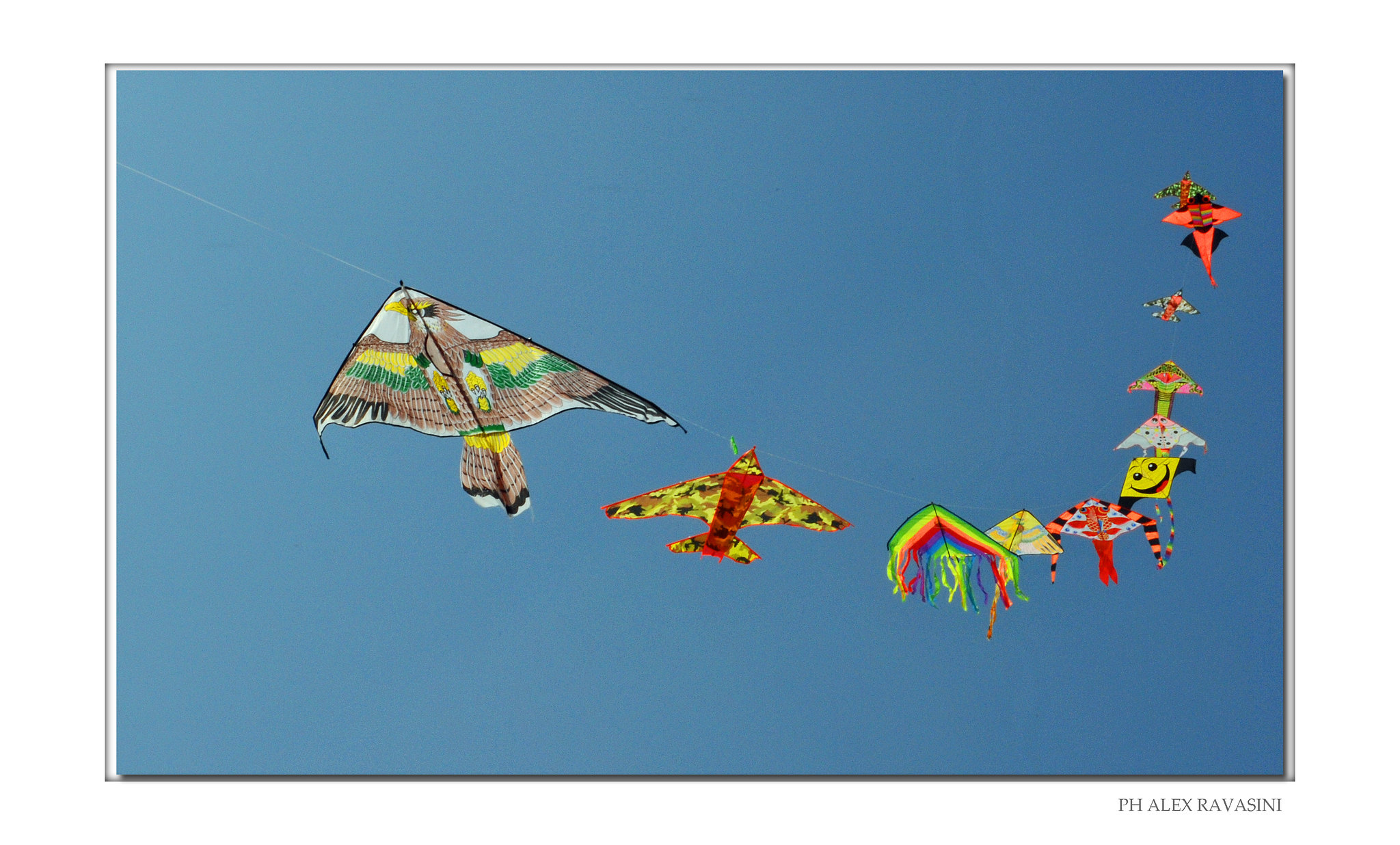In this vivid image of a clear blue sky with no clouds, we see an enchanting array of about eleven kites soaring high, tethered together in a u-shape formation. The kites vary in color and design, creating a captivating visual spectacle. Dominating the grouping is a bird-shaped kite with intricate brown, black, and white patterns, featuring an eagle's face with a yellow beak pointing to the left. Nearby, a red and yellow airplane-shaped kite adds a touch of whimsy. Further along the string, a rainbow kite with green fringe dances in the wind. There's also a vibrant assortment of other kites: a striking blue and yellow one, a multicolored kite with red, white, orange, and black hues, a cheerful yellow smiley face kite edged in black, a sleek white triangle kite, a green triangular kite with a matching tail, and two orange kites that complete the ensemble. These kites collectively form a mesmerizing chain against the pristine blue backdrop, though the individuals controlling them remain out of sight.